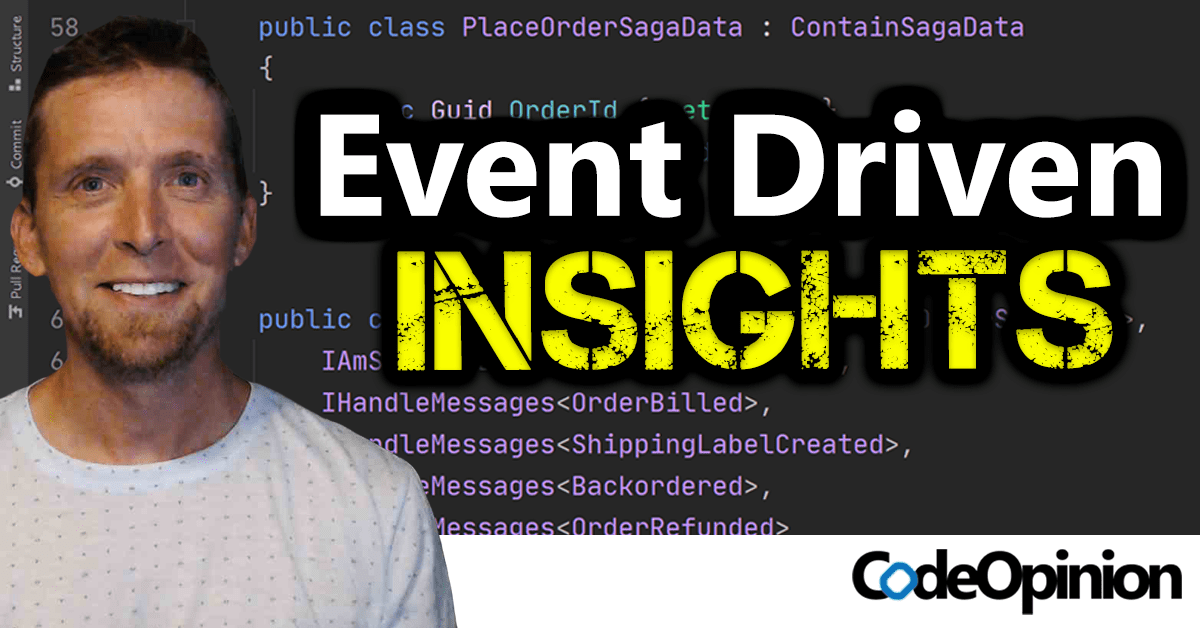This image captures a display ad designed within a rectangular frame featuring a medium to dark gray background. The background consists of a snippet of code from a webpage, characterized by syntax highlighting where "public class" is in blue, while "placeOrderSagaData" is prominently in purple.

On the left side, there's a headshot of a smiling white man in his mid-30s with reddish-brown hair and a beard. He wears a gray T-shirt adorned with subtle, slightly darker gray polka dots, giving it a textured appearance. His friendly demeanor and direct gaze towards the camera add a personable touch to the ad.

The central focus, however, is the headline to the right of the man and superimposed over the code background. It reads "Event Driven Insights," where "Event Driven" is in white and "Insights" is in yellow, both outlined in black for enhanced visibility.

At the bottom right corner, a white background segment contains the text "CodeOpinion," stylized as one word with a capital 'C' and 'O.' Notably, the 'O' in "code" is highlighted in blue, providing a distinct and cohesive branding element.